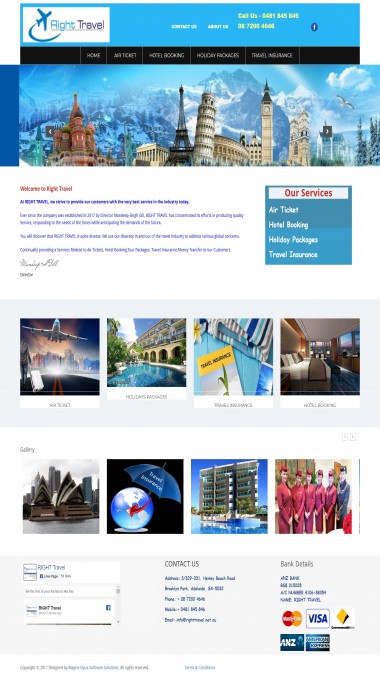This image captures a section of a travel agency's webpage. At the top of the webpage, the banner prominently displays the agency name, "Right Travel," accompanied by an airplane graphic soaring above the word "Right." Adjacent to this, there are navigation links such as "Contact Us" and "About Us." Additionally, a call-to-action in yellow reads "Call Us," followed by a phone number, also highlighted in yellow. 

To the right, there's an icon directing users to the agency's Facebook page. Below this, the main section of the webpage features an impressive montage of famous landmarks including the Leaning Tower of Pisa and the Eiffel Tower, set against a backdrop of majestic mountains and cloud-streaked skies.

Towards the middle right of the page, a dedicated box titled "Our Services" lists the travel offerings: air tickets, hotel bookings, holiday packages, and travel insurance.

Further down, the webpage showcases two rows of images, with four in each row, presumably highlighting various travel destinations or packages. At the bottom of the page, there is a "Contact Us" section, alongside bank details. Additionally, icons for accepted payment methods are displayed, including MasterCard, Visa, and American Express.